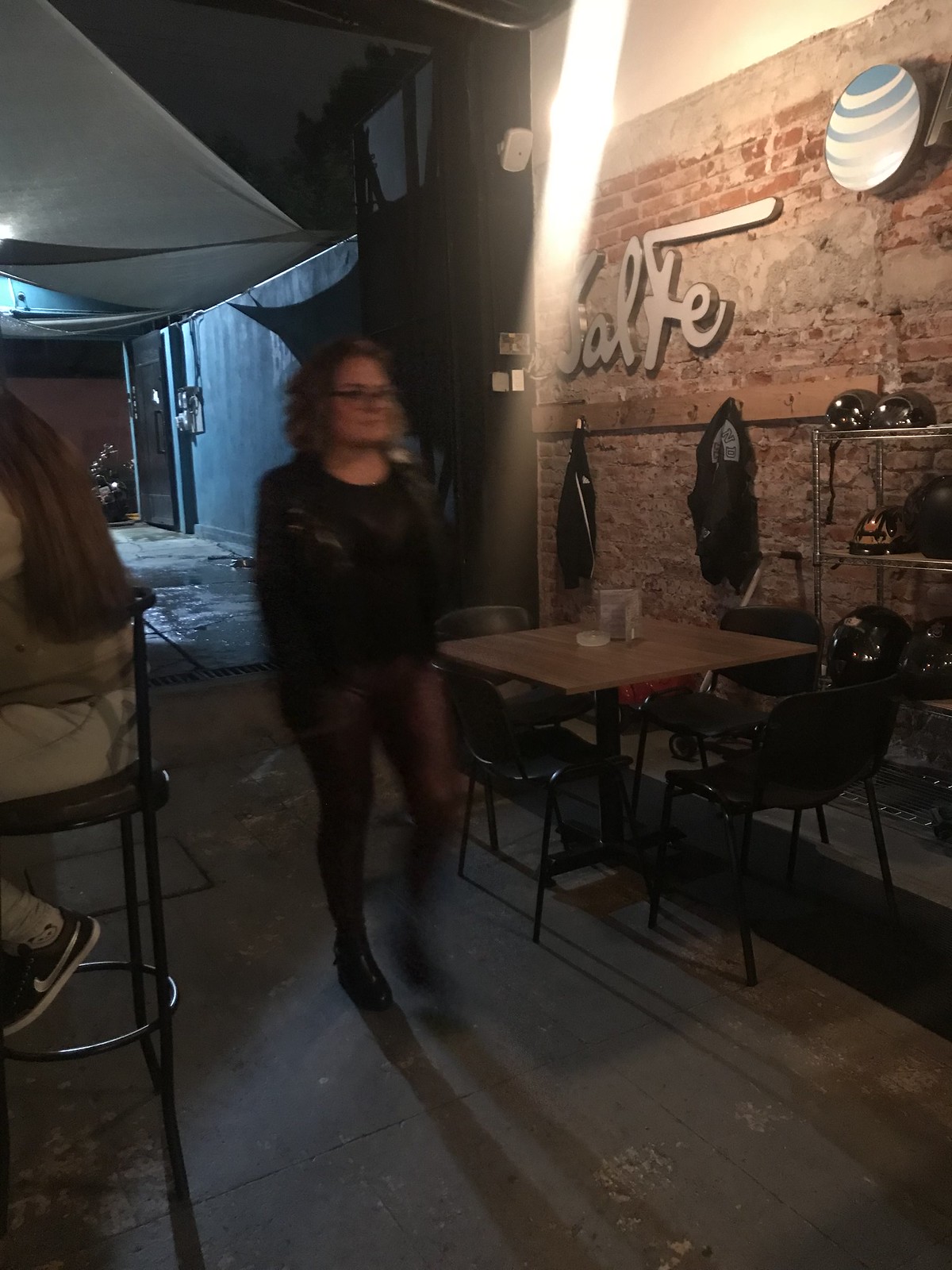In this rectangular photograph, we are presented with the interior of a bar or restaurant featuring an open patio area. Central to the image is a brown table accompanied by four chairs, on which stands a glass candle holder and a small, upright menu. The scene is bordered on the right by a brick wall adorned with the word "SALTE" in cursive script. Adjacent to the wall is a wooden rack equipped with hooks for hanging jackets. To the right of this, a three-shelf unit constructed of stainless steel or chrome displays several helmets.

On the left side of the image, we observe the profile of a man seated on a black bar-height chair, facing to the west. His upper body is partially out of frame, leaving his head unseen. In the center, a blurry figure of a woman is captured walking into the setting, facing forward as she enters.